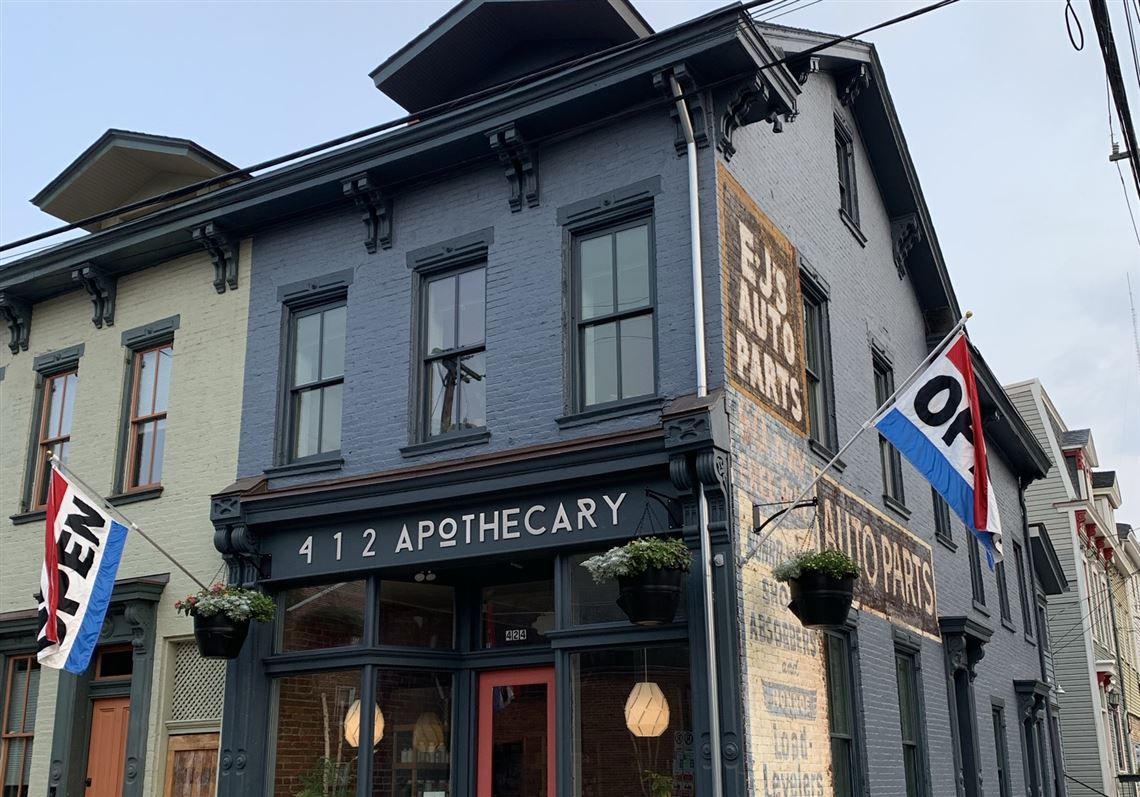This photograph showcases a historic, Italianate-style corner building with a shed hip roof, featuring two distinct storefronts. The building predominantly appears dark blue and is divided into an apothecary on one side and an auto parts store on the other. The apothecary at the forefront displays a sign reading "412 Apothecary" in contemporary font across a banner lintel. You can see two modern hanging globe lights giving off a soft glow, framing the red and black door. Alongside, two vertical flags indicating the store is open, each striped red, white, and blue with "Open" written in black, are displayed on either side of the apothecary storefront. On the second story of the building, to the left of the corner, there is another signless storefront. Around the corner, the side of the building reveals another storefront, identified by the pink sign "EJ's Auto Parts." Hanging plants add a touch of greenery to the building. The surrounding architecture features row houses reminiscent of those found in European towns or San Francisco, suggesting a historical district.